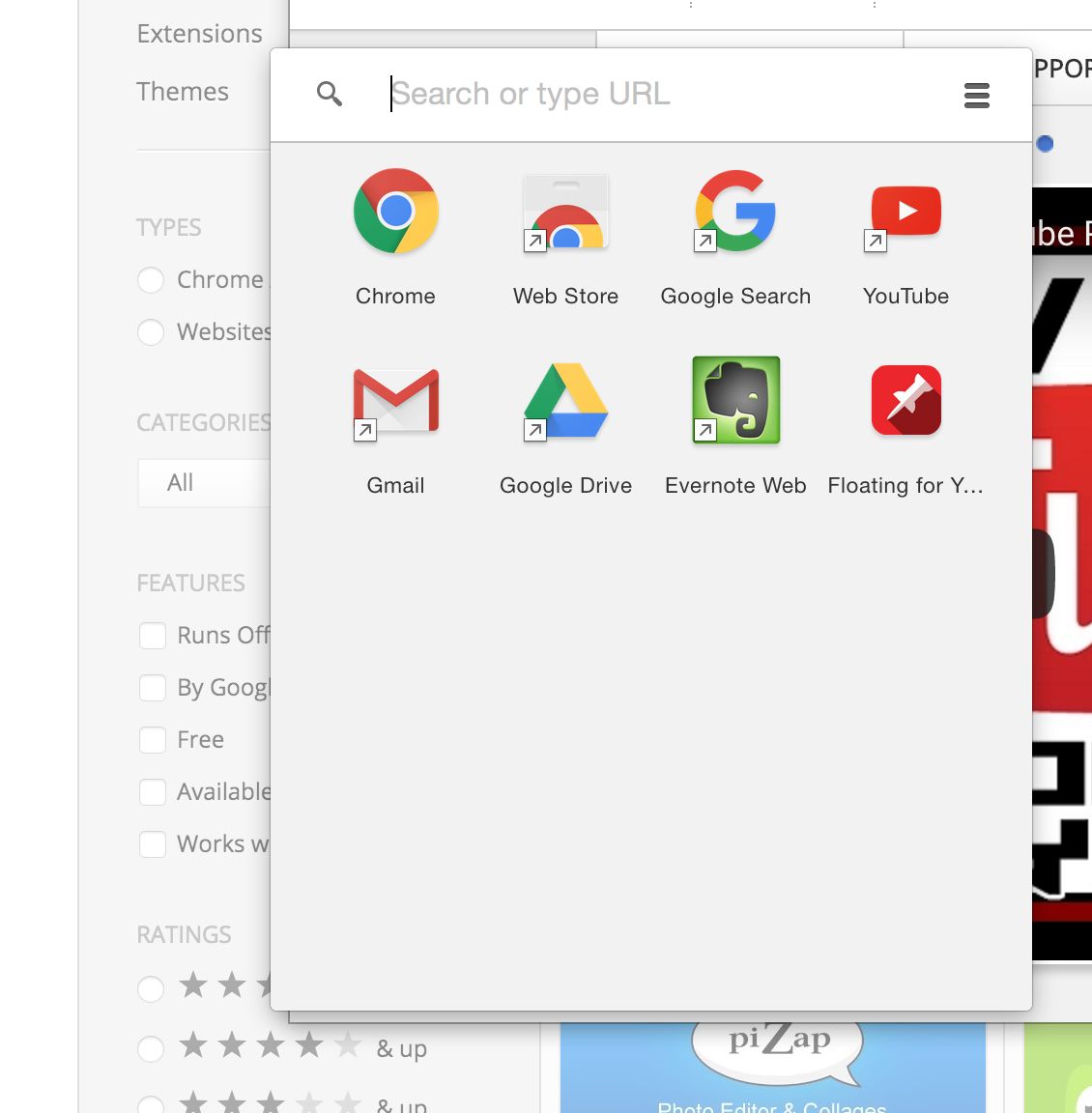The image appears to be a screenshot from a website, displaying a pop-up box in front of a partially visible web page. The background of the web page on the left is light grey, featuring a panel with a list of words such as "extensions," "themes," "types," "chrome," "websites," "categories," and "all features" in dark grey. Further down the panel, there are options to filter content, including "run off by Google," "free," "available," "works with," and selections for ratings.

To the right of this panel, partially visible images in red seem to represent YouTube videos, contrasted with the site's red, black, and white color scheme. Below, there is a blue background featuring a speech bubble labeled "PZAPP," with something green situated at the lower right corner.

The focus of the screenshot is the pop-up box. It has a white bar at the top, housing a search icon and a search input field labeled "Search or type URL." At the far right of this bar is a hamburger menu icon. Below the search bar, on a very light background, there are two rows of various app icons.

The top row consists of icons for Chrome, Web Store, Google Search, and YouTube. The bottom row includes icons for Gmail, Google Drive, Evernote Web, and another app, only partially labeled and denoted by a pin with a red background. The last visible icon in this row has an incomplete label reading "Y..." dot dot dot. The design of this pop-up box, with its search bar and list of app icons, suggests an interface that might be unfamiliar or unconventional for the typical user.